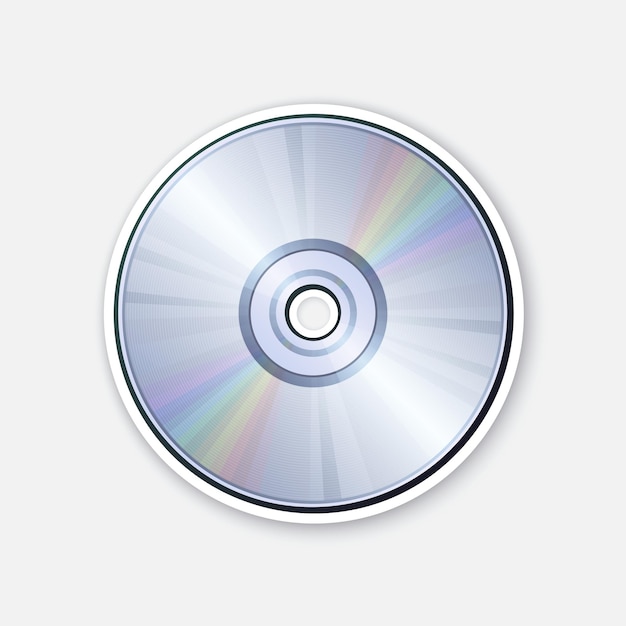The image depicts a computer-generated, overhead view of a blank CD or DVD, centered on a white background. The disc rests on a CD holder with a central column. The CD’s design features a series of concentric rings with alternating colors and textures. The outermost border is a white ring, followed by a black ring, a raised blue border, and then a gleaming silver section. The center area features several rings of varying shades of gray and black, including dark gray, light gray, and black, with subtle transitions between them. The outer edges display a rainbow pattern due to polarized lighting effects. The CD's surface is new and shiny, with both rainbow and white light reflections adding to the visual complexity. The clear center hole allows the white background to be visible through it.